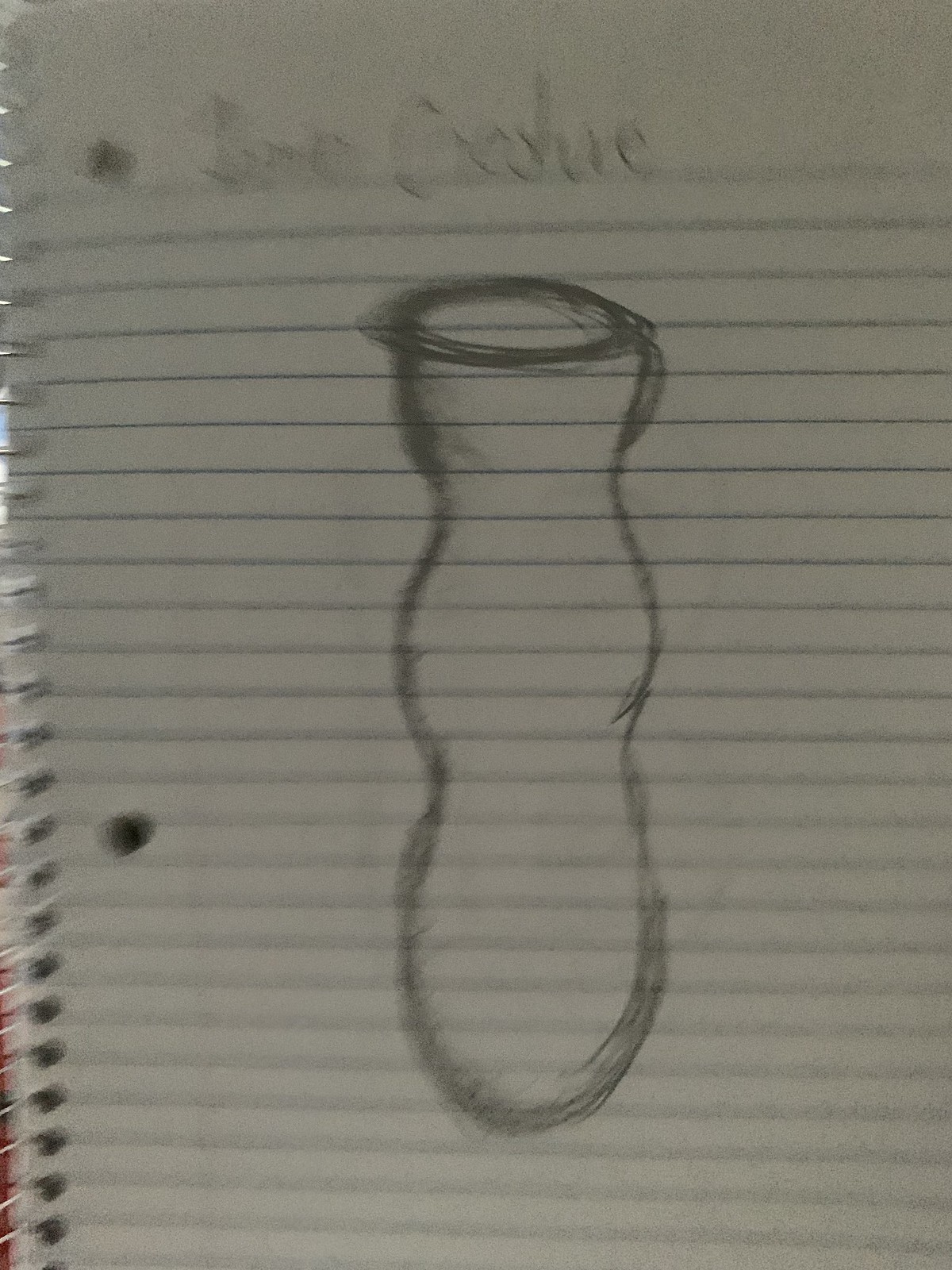This is a photograph depicting a slightly blurred and grainy close-up of a notebook page. The page, with clearly visible horizontal lines, appears to be spiraled off to one side. At the top of the paper, there is some handwritten text in pencil, although the low image clarity renders it illegible. Dominating the page is a pencil drawing that resembles a tornado, characterized by intense scribbling, especially concentrated at the top, suggesting multiple strokes or revisions. The rest of the page is blank with no additional drawings or text. The background of the image is devoid of any other objects.